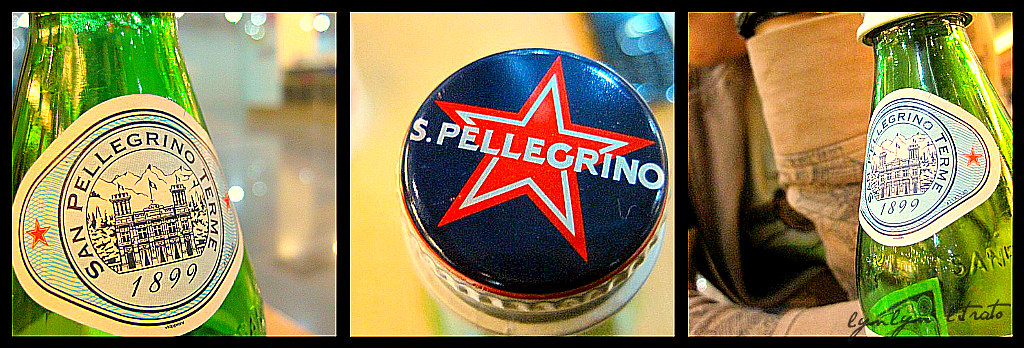The image is sectioned into three professionally lit, close-up photos of a San Pellegrino Terme 1899 bottle, each separated by a black border. The leftmost square features a detailed view of the label, showcasing its green bottle, adorned with red stars, blue lines, and a central circle encasing an illustration of a building, with “San Pellegrino Terme 1899” prominently displayed. The middle square presents a top-down shot of the bottle cap, which is blue and bears a red star encircling a smaller white star, and the words “S Pellegrino” in white lettering. On the right, the image captures another angle of the green bottle, showing both the label with its intricate logo and the cap with the previously described details. The bottle appears to be empty, and the signature "Lynn Lynn" is visible at the bottom of the label.